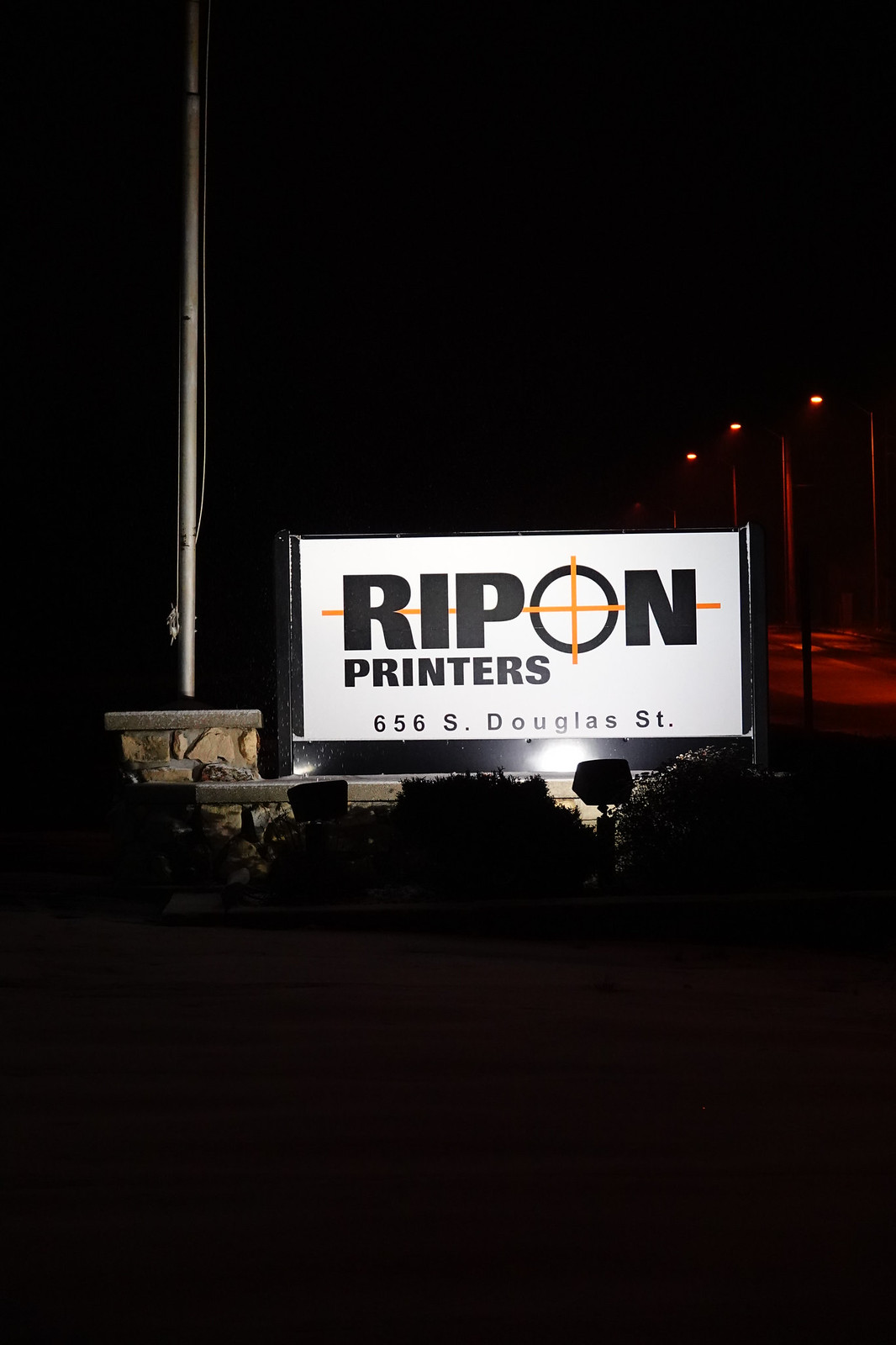The image, taken at night, features a prominently lit white sign with a black border that reads "Rip On Printers, 656 S Douglas Street." The "O" in "Rip On" is distinctively designed as an orange crosshair. This sign is perched atop a low brick wall and is illuminated by ground-mounted floodlights. To the left of the sign, there is a brick base supporting a silver flagpole, which stretches diagonally from the middle-left to the top-left of the image. In the background on the left, faintly visible, are three streetlights and a street area bathed in a red glow. The foreground shows some dark pavement and the shadowy outlines of bushes beneath the sign. Above the sign, the sky is entirely black, emphasizing the nighttime atmosphere.